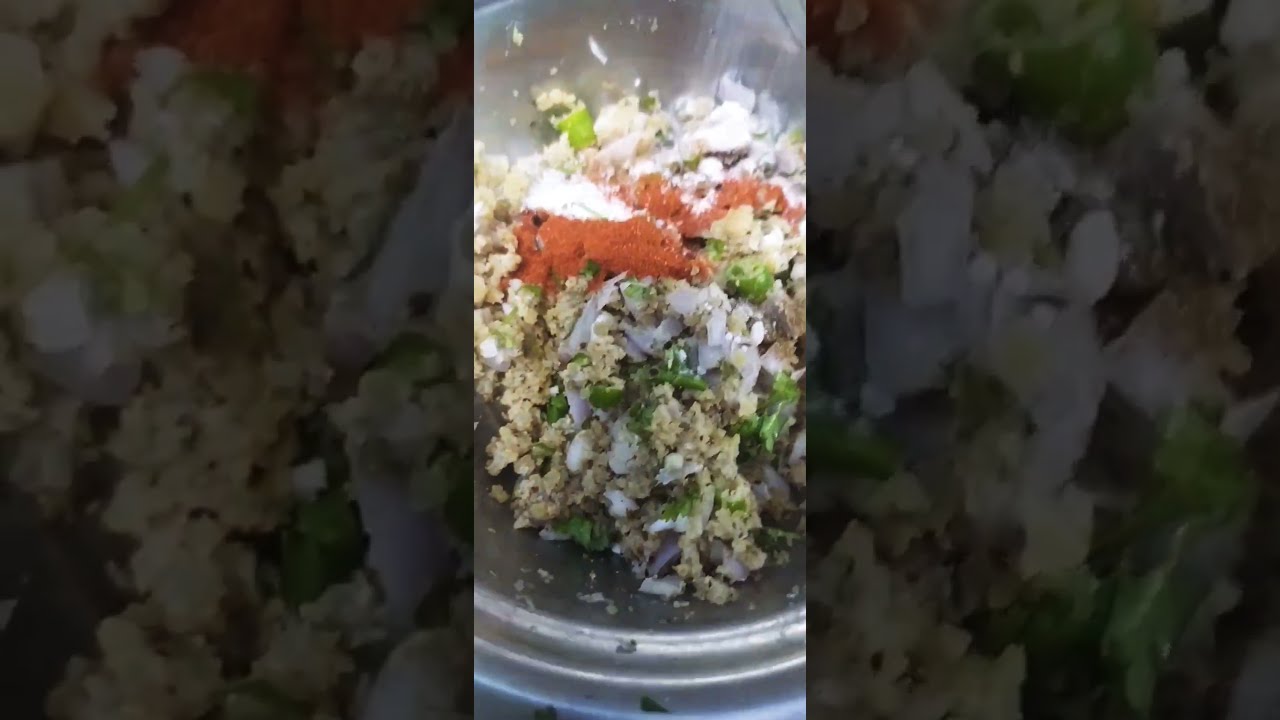The image depicts a mixed salad being prepared in a silver or metal bowl. The contents include various ingredients such as rice, possibly brown and cooked in olive oil, imitation or real crab meat, and diced green vegetables which might include celery, green peppers, spinach, or asparagus. There are also likely some cut mushrooms and small white pieces which could be onions, as well as red onion fragments. A powdery red substance, probably paprika, is sprinkled on top. The salad features a mix of green herbs, tomatoes, and couscous or similar grain. The photograph appears in the center of the frame as a clear vertical rectangle, flanked on either side by a blurry, zoomed-in, and darker version of the same image, suggesting it might be a screenshot from a video.